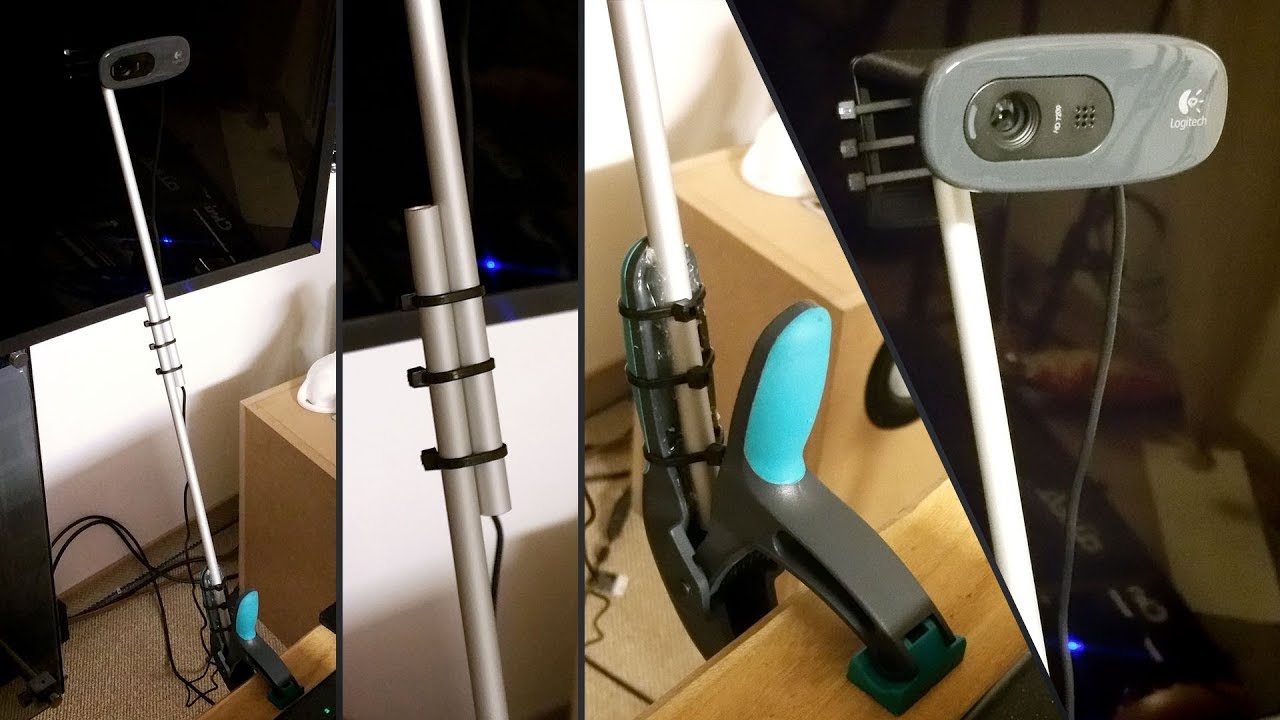The image collage consists of four photographs that detail a setup involving a webcam mounted on a pole. The leftmost photograph provides a full view of the entire assembly: a Logitech webcam, which has an oval shape and a mix of gray and black colors, mounted at the top of two metallic poles. These poles are joined together by three black zip ties in the middle and are further secured to a vise grip at the bottom using three additional zip ties. The vise grip, which is black and blue, is attached to a desk. The background features a white wall and a window, with a tan carpet on the floor, and a tan shelf visible in the lower right corner. The second photograph from the left zooms in on the two poles connected by the zip ties. The third image offers a close-up of the vise grip clamped to the desk. The rightmost photograph provides a close-up of the Logitech webcam mounted atop the poles, highlighting the zip ties used for securing it.